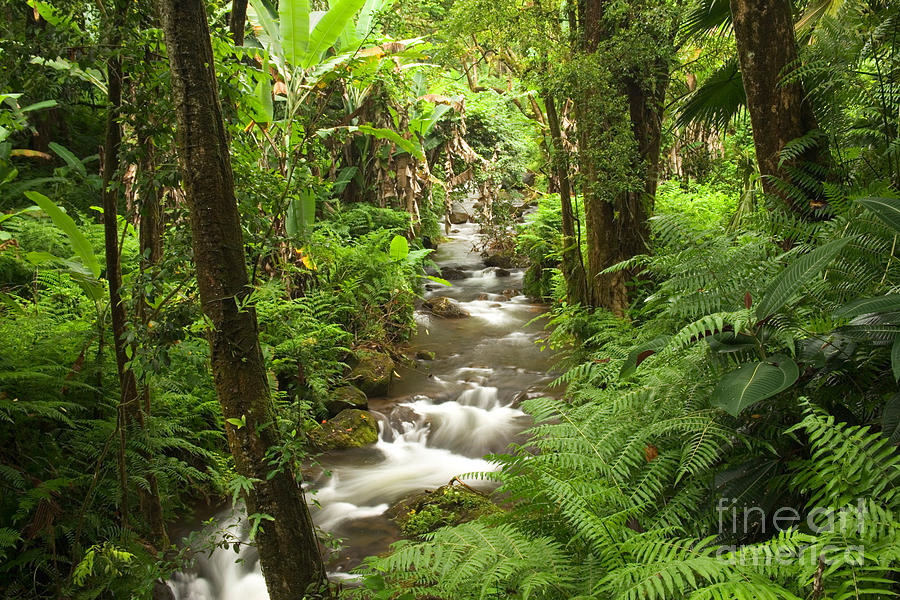The image, potentially created using CGI or captured with a highly detailed and focused lens, portrays a lush jungle landscape in landscape orientation. Dominating the scene is a winding creek that descends from the middle top of the image and curves to the left just before reaching the bottom of the frame. The stream, white and frothy in places, flows past moss-covered rocks which dot its edges and even appear within the water itself. Surrounding the creek is a dense array of green vegetation, including thick ferns, some moss-covered trees, and possibly banana trees. A prominent tree rises from the bottom left, extending out of view at the top left. More trees, equally tall, frame the right side of the image, amidst a profusion of green growth. In the bottom right corner, faint white or gray text reads "Fine Art America," adding a discreet signature to the vibrant, verdant scene. The intricate details and dynamic water flow suggest digital enhancement, giving the impression of a moment captured in vigorous motion.